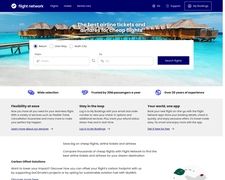The website features a striking image of a mountainous landscape. Prominent, snow-capped peaks rise majestically against a crystal-clear, vibrant blue sky. Nestled at the base of these towering mountains is a quaint village, its buildings rendered in shades of brown and white, evoking a serene alpine charm. A tranquil lake sits at the foot of the mountains, mirroring both the imposing peaks and the cozy village in its reflective waters.

At the top of this website is a dark blue-purple header, adorned with white text. Just below this header, three sections of text are displayed, though the font is too small to discern specific details. In the picturesque scene, lush greenery punctuates the landscape, with evergreen trees adding a splash of verdant life. The mountains themselves are portrayed in earthy browns, topped with sparkling white snow caps.

Further down the webpage, a gray box containing three paragraphs of text spans across the page, likely providing more information about the featured area. Beneath this gray section is a white box with additional text. To the lower right, a green graphic with dotted embellishments adds a touch of modern design elements to the overall page layout.